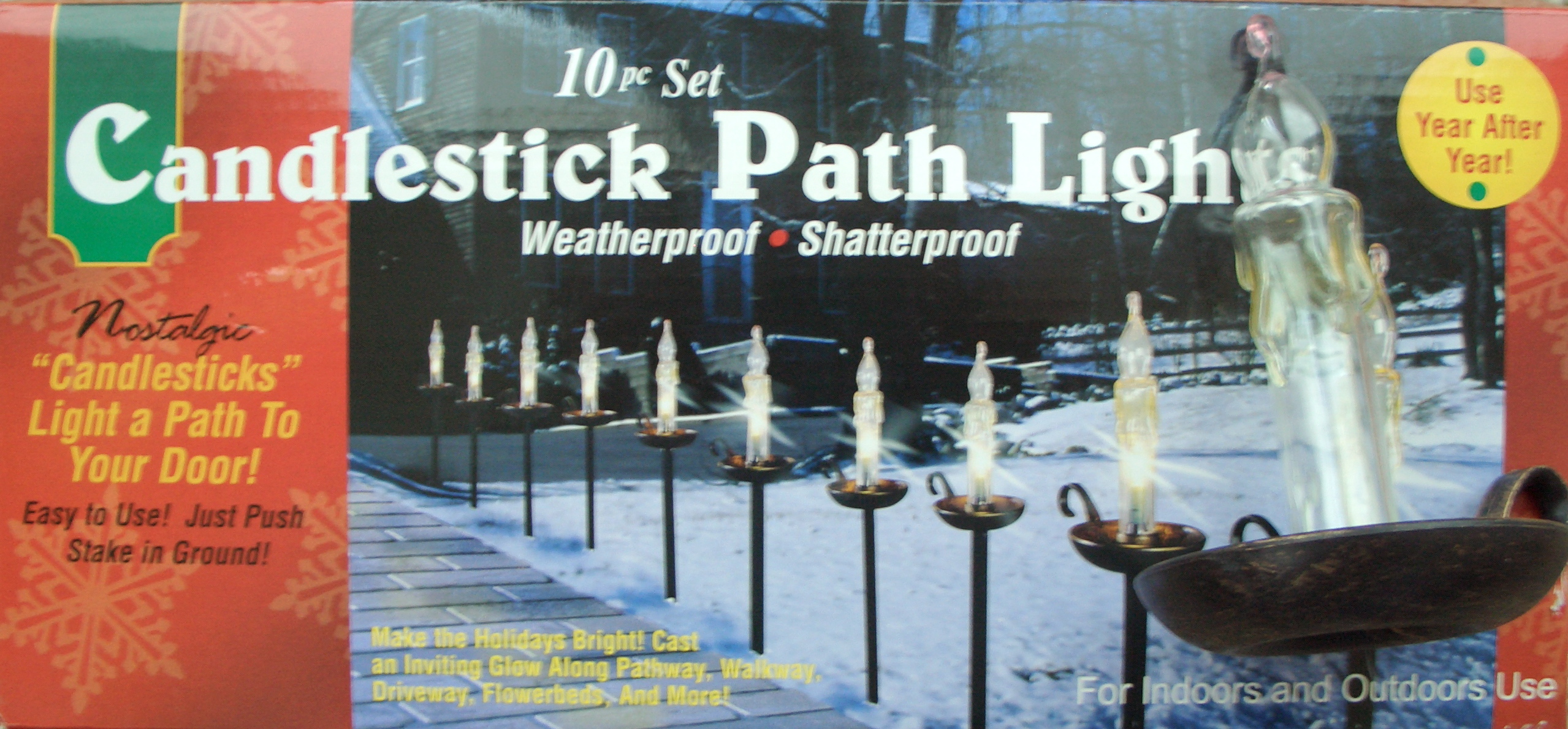The image shows a close-up of an old-fashioned magazine cover or product box featuring a "10-piece Candlestick Path Light" set. The set includes nostalgic, electric candles designed to look like traditional candlesticks with metal bases and plastic tops, mimicking the appearance of candles with little bowls and handles. These lights are described as weatherproof and shatterproof, suitable for both indoor and outdoor use. The description emphasizes their durability and ease of use—simply push them into the ground to light a path, driveway, flowerbed, or waterway. The packaging details that these lights are perfect for making the holidays bright by casting an inviting glow along pathways. The image on the box illustrates the candles lining a snowy walkway leading to a house in the background.